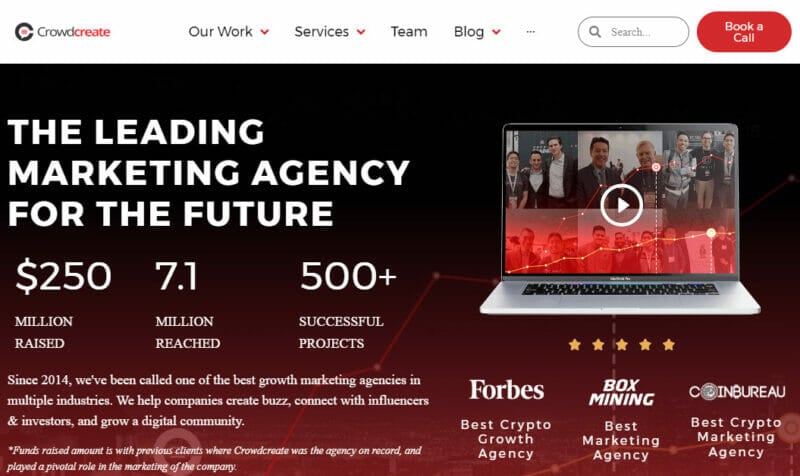In the image, the header section on a white background prominently features the brand name "Crowd Create" on the top left, where "Crowd" is in grey and "Create" is in red. An icon of a black "C" with a red dot inside accompanies the brand name. The navigation bar includes drop-down menus labeled "Our Work," "Services," "Team," and "Blog." To the far right of the header, there is a search bar and a red "Book a Call" button with white text.

Below the header, on the main body of the page, the right side contains the tagline "The Leading Marketing Agency for the Future" in white text. Key achievements are highlighted underneath: "$250 million raised," "7.1 million raised," and "several successful projects."

The bottom left section states: "Since 2014, we have been recognized as one of the best growth marketing agencies in multiple industries. We help companies create paths, connect with influencers and investors, and grow a digital community. The fund raised amount is from previous campaigns where Crowd Create was the agency on record and played a pivotal role in the company’s marketing efforts."

On the right side, there is an image of a white laptop displaying a video that features market growth lines with people faintly visible in the background. The laptop's play button is white. 

Towards the bottom, a 5-star rating is shown with yellow stars. The text below it reads, "Forbes: Best Crypto Crowdfunding Agency," "Box Mining: Best Marketing Agency," and "Coin Payroll: Best Crypto Marketing Agency," in white text. The background is split: black on the top half and red on the bottom half, which also features red lines symbolizing market fluctuations.